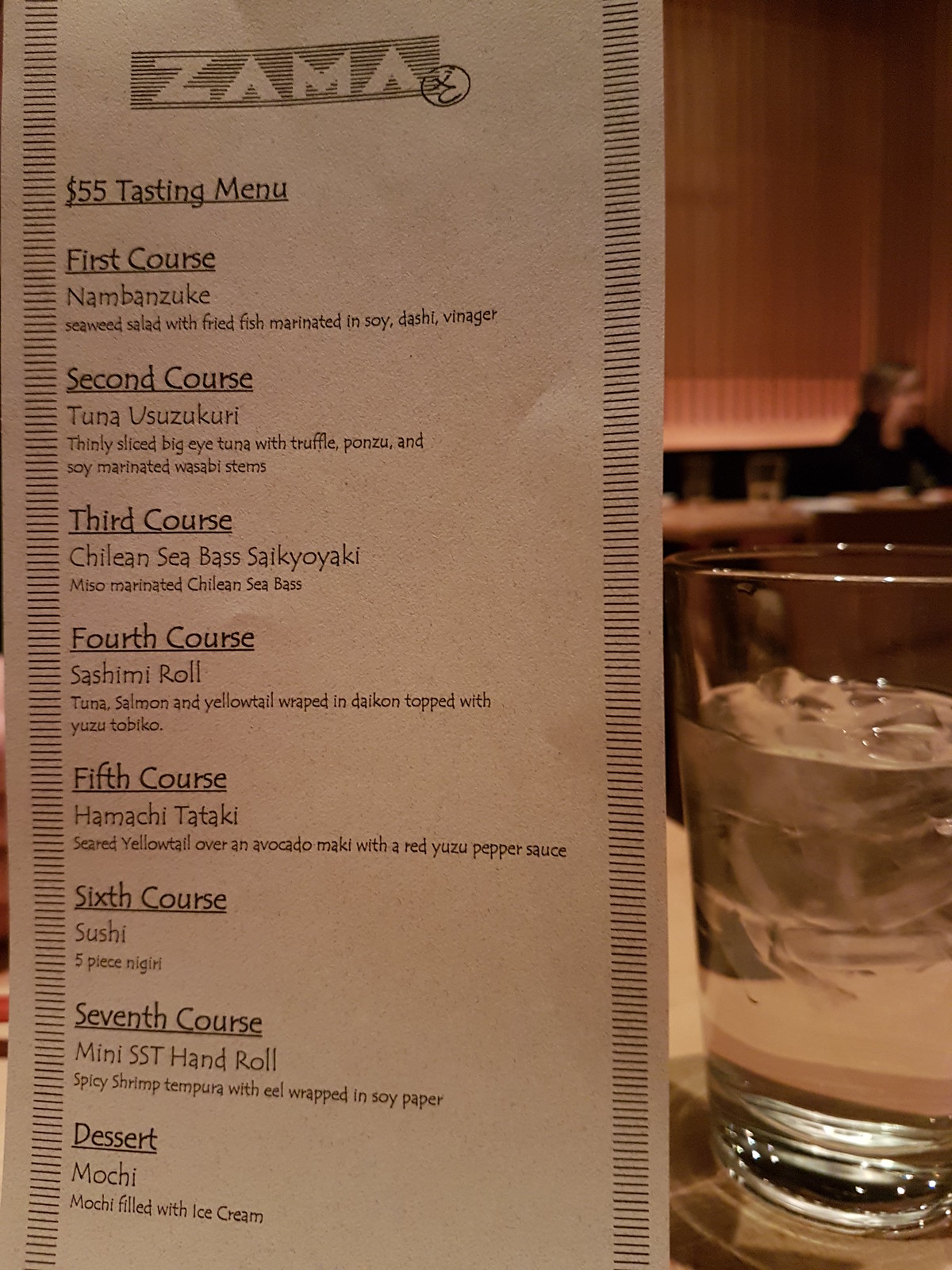This image showcases an elegant tasting menu from ZAMA. The menu's title, "ZAMA," is prominently displayed at the top in a light gray color against a dark gray background, with the A's stylized as triangular tent shapes. Beneath the title, the menu introduces a "$55 Tasting Menu" in bold black text. The entire menu features black text on a light gray backdrop, highlighting each course in a clean, organized manner.

The courses are listed sequentially:
- First Course
- Second Course: Tuna Usuzukuri (beneath which is some explanatory text)
- Third Course
- Fourth Course
- Fifth Course
- Sixth Course
- Seventh Course
- Dessert

The menu design includes very thin, dark gray horizontal lines running vertically along the left and right edges, adding a subtle, sophisticated touch.

To the right of the menu, a glass of water, filled three-quarters of the way with ice, is visible. In the background, an individual dressed in a black jacket is seated at a table, creating a sense of dining ambiance. The wall behind the individual is a dark brown color, contributing to the image's overall warm and inviting atmosphere.